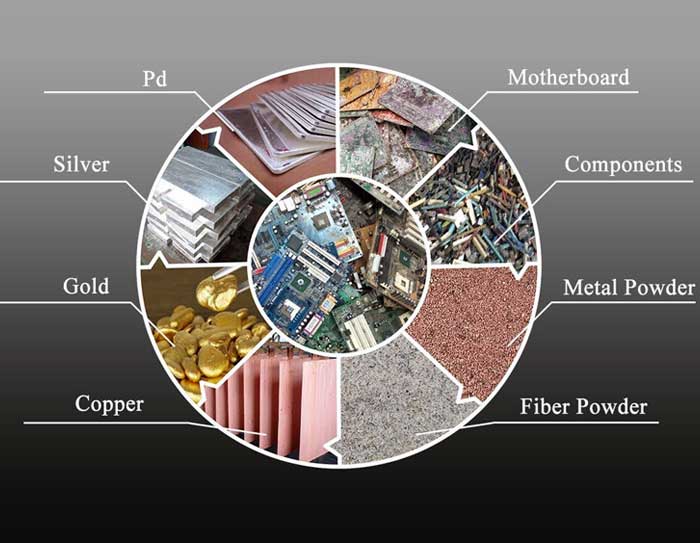The image is a detailed infographic that fuses photographic elements with graphic design and typography. Centrally, there is a circle filled with a photograph showcasing heaps of microchips, displaying shades of grays, blues, and greens. This central circle represents the core of the diagram. Surrounding it, the image transforms into a pie chart divided into eight sections, each meticulously labeled with white lines pointing to its respective pie slice. 

Starting at the top right and moving clockwise, the sections are labeled as follows: motherboard, components, metal powder, fiber powder, copper, gold, silver, and PD. Each of these labels is depicted in white text. The background of the image is an ombre gradient, transitioning from gray at the top to black at the bottom, adding depth and contrast to the illustration.

Each pie slice contains a colored photograph relevant to its label, visually representing the different materials and components such as powders, metals, and electronic parts. The exterior of the pie chart is outlined with a white line, ensuring a clear and crisp separation of each section. The overall style combines photographic representationalism with modern graphic design, making it an informative and visually engaging illustration of microchip components.